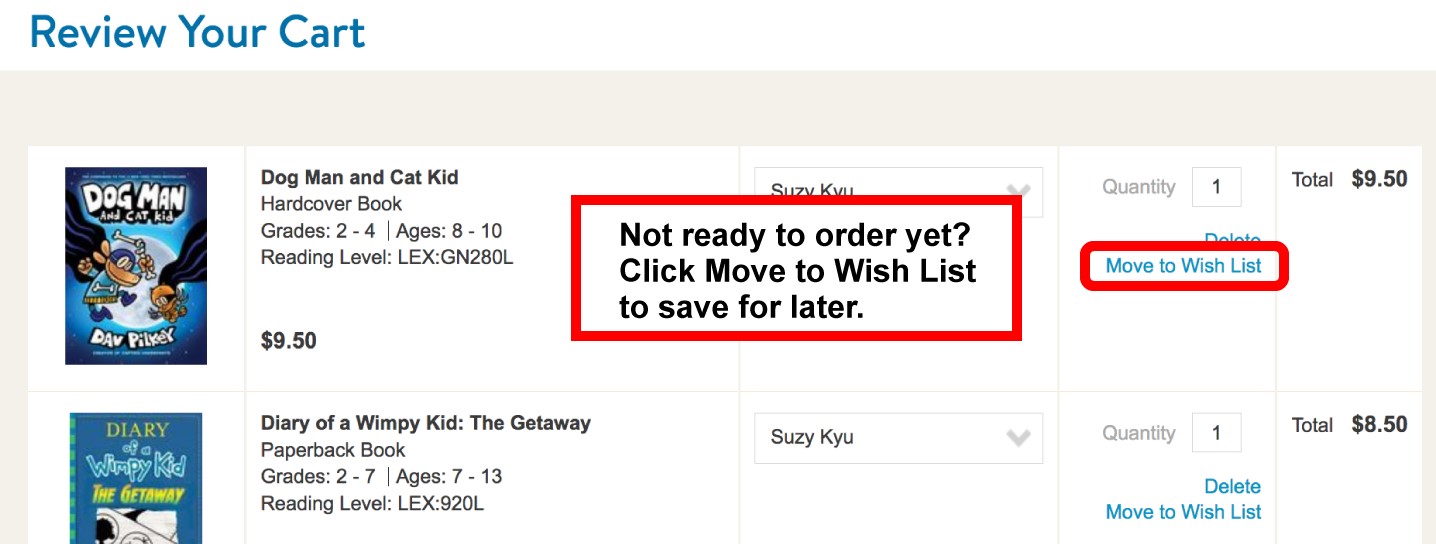**Descriptive Caption:**

The image depicts a cropped screenshot of a "Review Your Cart" page from an online store. The uppermost portion of the image features a prominent blue text in the largest font on the page, reading "Review Your Cart" against a white background. Directly below this, the background shifts to light gray, within which is a smaller, central white box containing the cart details.

Starting from the left of the white box, there is a tall rectangular image resembling a book cover preview, titled "Dog Man and Cat Kid." The illustrated cover features characters dressed in capes. Adjacent to the book cover, to the right, the product information is listed: "Dog Man and Cat Kid, Hardcover book, Grades 2-4, Ages 8-10." Below this is an additional specification, "Reading level: LEX GN-280L."

Overlaying part of this product information is a noticeable black text message that reads, "Not ready to order yet? Click 'Move to wish list' to save for later." This message is outlined with a red rectangle drawn by the user. The outline partially obscures the name "Suzy Kiyu," which appears in the product information, and another row beneath shows the same duplicated details. Also visible is the product quantity of "1" and the price "$9.50." A red rectangle highlights the blue text link "Move to wish list," and it slightly covers the word "delete."

Beneath this entry, the second row features another book, "Diary of a Wimpy Kid: The Getaway." The book cover image is not fully visible, with approximately 70% shown. To its right, similar detailed product information is provided: "Diary of a Wimpy Kid: The Getaway, Paperback book, Grades 2-7, Ages 7-13, Reading level: LEX 920L," followed by "Suzy Kiyu" and a "V" symbol in the subsequent columns. The quantity is listed as "1," with a total price of "$8.50," alongside links for "delete" and "Move to wish list."

This elaborate breakdown captures the entire visible content of the cropped screenshot image.